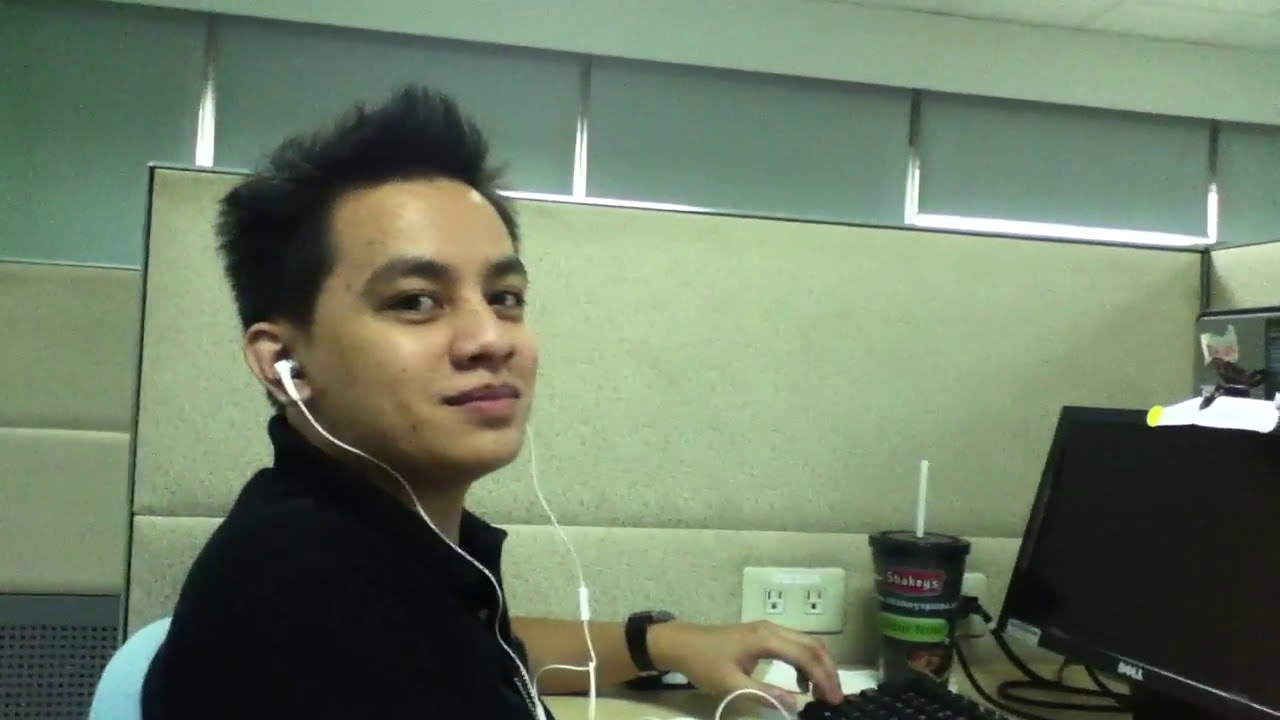The image captures a young Asian man, possibly in his 20s or early 30s, seated sideways in an office cubicle but looking directly at the camera with a slight, friendly expression. He has earbuds in his ears and is dressed in a black shirt, wearing a black watch. The cubicle features a silver Dell computer screen in the bottom right corner, which is off and dark, along with a keyboard in front of him. There is also a large cup with a straw, likely containing coffee, placed next to an exposed power outlet. The cubicle walls have a white fabric texture, and the background shows closed windows, indicating it's an indoor setting with likely artificial lighting.